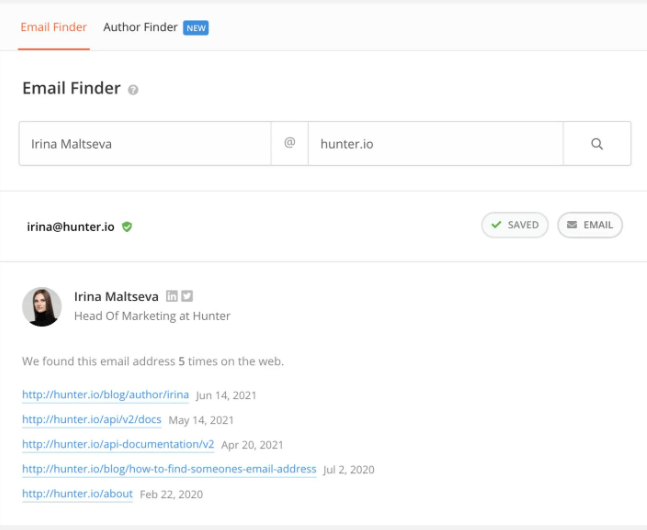Here is an image caption based on the provided description:

---

A screenshot of a website interface showcasing an email finder tool. The layout is minimalist with a predominantly white background. At the top of the screen, there are two main options: "Email Finder" in red lettering with an underline slightly below the text, and "Author Finder" with a "new" symbol next to it. Just beneath this section, "Email Finder" is displayed again accompanied by a small question mark inside a circle for additional information.

Below this header, there are two input fields. The first field defaults to the name "Irina Maltseva" and includes an "@" symbol towards the right. Connected to this is another defaulted input section that reads "hunter.io" with a search icon at the far right. Below the inputs, the email address "Irina@hunter.io" is shown with a green checkmark indicating its verification status.

To the left, there is a headshot of a woman labeled "Irina Maltseva," followed by her title, "Head of Marketing at Hunter." The page notes that this email address has been found five times online, and lists five corresponding URLs with HTTP addresses in blue text, each slightly underlined and accompanied by dates on the right.

---